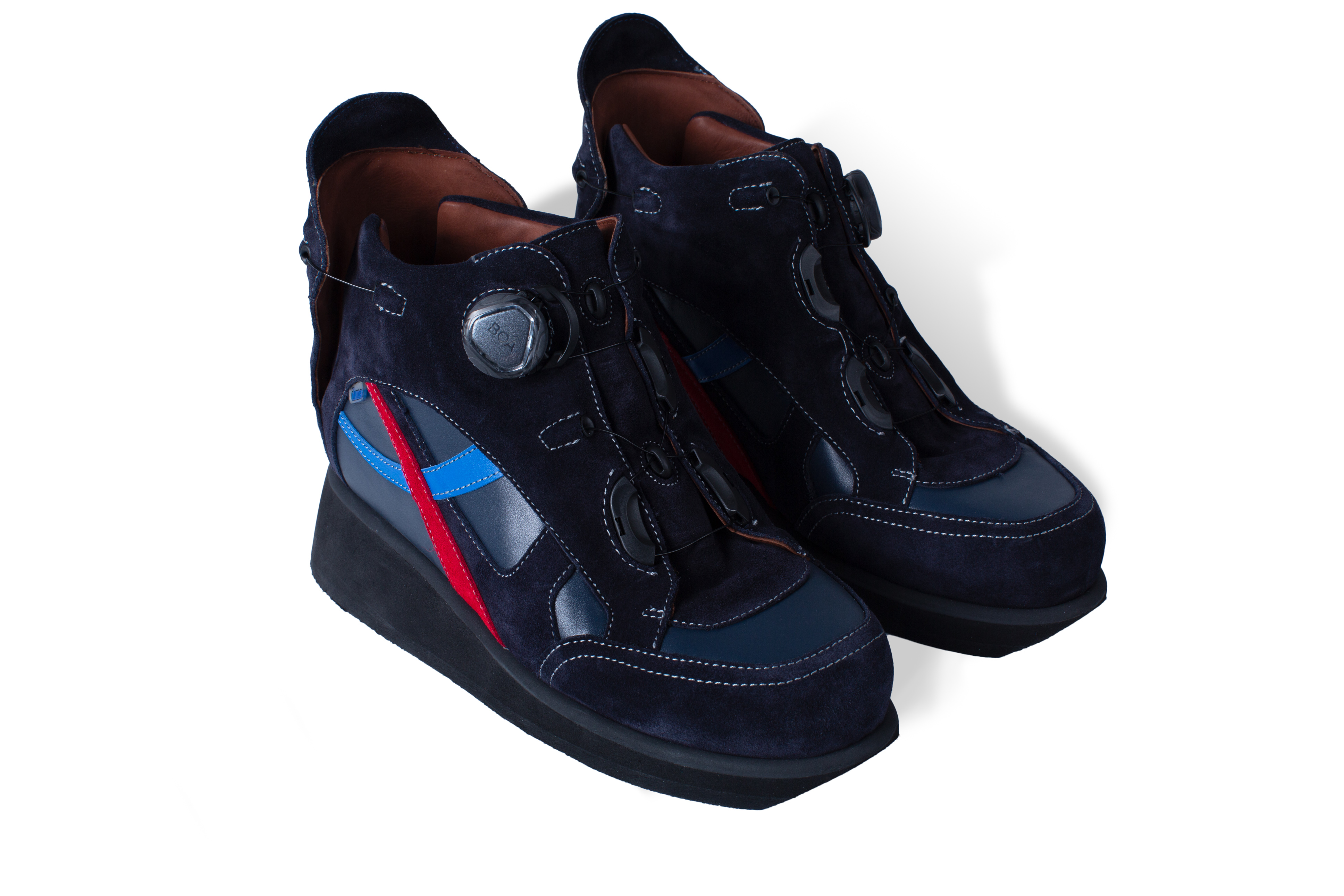This detailed photograph showcases a pair of sleek, high-tech children's boots set against a contrasting black and white background. The boots, which are small and velvety black with high platforms, are equipped with intricate details that highlight their unique design. A prominent feature includes a large, triangular-shaped button on the top. They boast a combination of black leather front panels intersected by a striking red and blue stripe pattern along the sides, forming an 'X' shape. Despite their futuristic and somewhat clunky appearance, the boots forsake traditional laces and instead use advanced, high-tech buckles at the front for fastening, alongside an adjustable heel area to ensure a snug fit. The inside part of the boots reveals a rich brown leather lining, and the white stitching stands out against the dark fabric, adding to the intricate design. The image casts a light gray shadow to the right, enhancing the dramatic look of these custom-made, multipurpose boots.